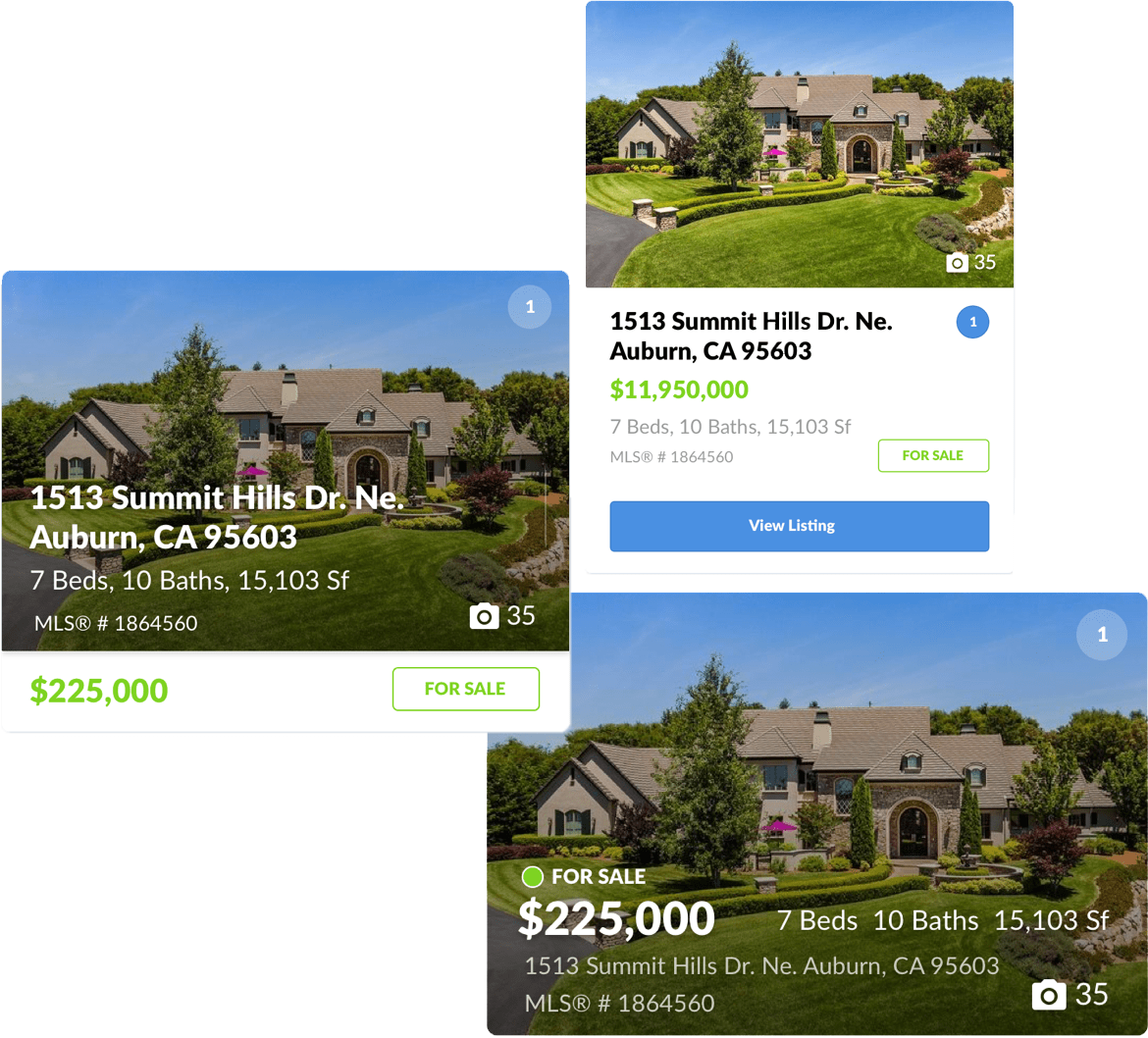This image showcases a stunning house listed at 1513 Summit Hills Drive in Auburn, California. The gallery comprises three images, all depicting the same house. One image includes a camera icon indicating that there are 35 photos available for this property. The house is a grand, two-story residence that appears to occupy a corner lot. It features excellent landscaping with lush green lawns and multiple trees in both the front and backyard.

The exterior of the house has a sophisticated grayish-brick color, complementing its beautiful window designs and an elegant arched doorway. The sky is a clear blue, enhancing the home's curb appeal. In one of the images, a purple umbrella can be seen in the backyard, adding a touch of color to the outdoor space. 

The property boasts impressive dimensions with 15,103 square feet of space, including seven bedrooms and ten bathrooms. It is listed for sale under MLS number 1864560. Initially, the house was listed at $11,950,000 but currently is shown with a significantly reduced price of $225,000, suggesting either a drastic price drop or a potential error in listing. The green "For Sale" button indicates its active status on the market. This home is not only expansive but beautifully designed and thoughtfully landscaped, making it a desirable property.